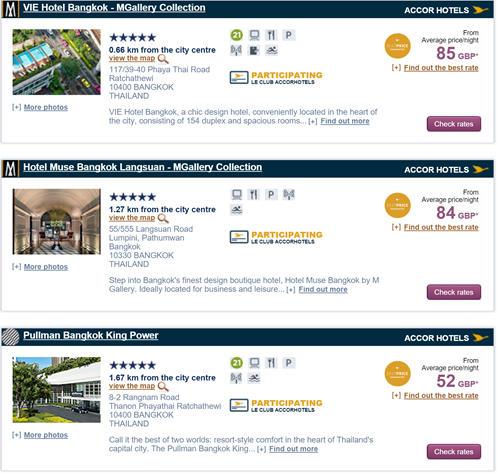Screenshot showcasing information about three luxury hotels in Bangkok within the M Gallery collection, featuring a clean white background. 

1. **VIE Hotel Bangkok M Gallery Collection**
   - Rating: 5 stars
   - Proximity: 0.66 KM from the city center
   - Price: £85 GBP
   - Features: Located in a highlighted orange section on the map with an orange magnifying glass icon

2. **Hotel Muse Bangkok - M Gallery Collection**
   - Rating: 5 stars
   - Proximity: 1.27 KM from the city center
   - Price: £84 GBP
   - Features: Positioned in an orange section on the map with an orange magnifying glass icon

3. **Pullman Bangkok King Power**
   - Rating: 5 stars
   - Proximity: 1.76 KM from the city center
   - Price: £52 GBP
   - Features: Indicated with an orange section on the map, featuring an orange magnifying glass icon

All hotel entries feature detailed information about their ratings, proximity to the city center, and pricing, each marked with a distinctive orange highlight for easy identification on the provided map.